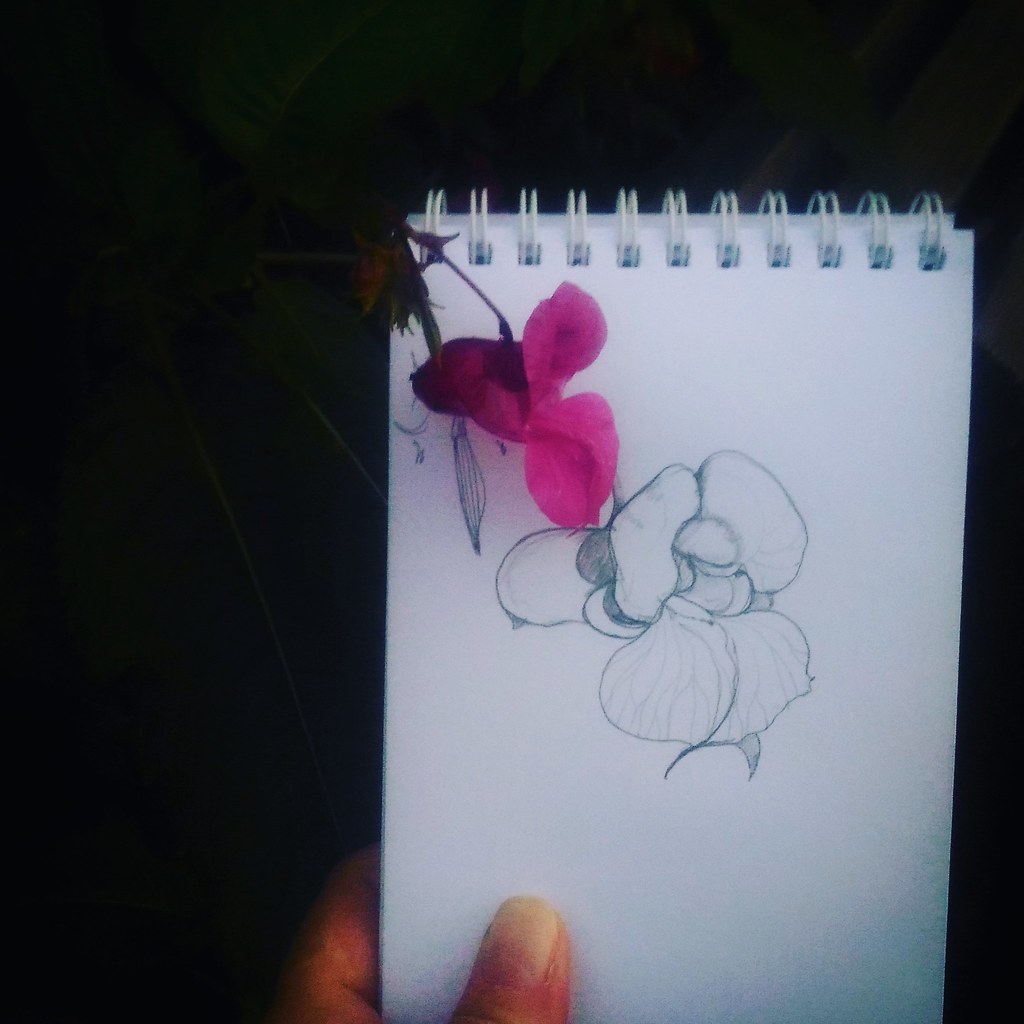In the photograph, a left Caucasian hand, with its thumb and index finger visible, holds up a white spiral-bound notepad with its pages in portrait orientation. The background of the image is entirely black, making the notepad stand out prominently. The spiral rings are positioned at the top of the notepad, which appears to contain white pages that can be flipped over. Attached to the top left corner of the notepad is a real, vibrant flower. While the exact color seems to vary between descriptions—being noted as purple, yellow, or pink—the flower has three main petals and is held in place by a green stem, possibly hanging over from the side. 

The notepad features a detailed pencil drawing of the flower, meticulously replicating its shape and details, including the center, petals, and some shading, indicating that the drawing was likely done by an adult. This thoughtful sketching attempts to closely mimic the real flower, suggesting that the person holding the notepad might have drawn it while observing the flower closely. The drawing, enhanced by careful shading and realistic lines, confirms the artistic effort put into capturing the flower's essence.